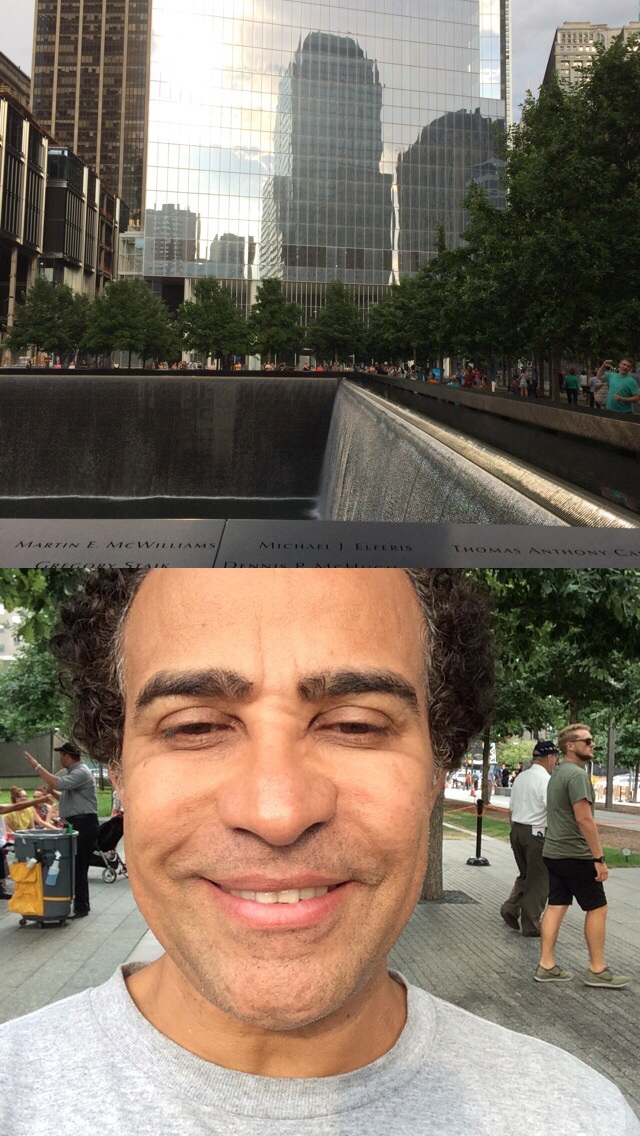The image is a two-part photo showcasing two distinct scenes. The top part features a bustling cityscape, likely New York City, portraying what appears to be the 9-11 Memorial. A massive building with clear, glass windows dominates the background, reflecting the surrounding skyline. Encircling a central fountain are numerous trees, their green leaves providing a stark contrast against the adjacent buildings with white facades trimmed in black. Scattered amidst this tranquil setting are people, emphasizing the memorial-like atmosphere with names etched into marble surfaces reminiscent of the Vietnam Memorial Wall.

The bottom part of the image captures a casual selfie of a middle-aged, light-complexioned African-American man. He has tightly curled brown hair with hints of gray, bushy eyebrows, and a five o'clock shadow. Dressed in a light gray shirt, the man exudes a mild smile. Surrounding him are everyday city scenes: a man to his left is pushing a trash can, possibly cleaning the area, while two casually dressed men stand to his right. In the background, further enhancing the casual city vibe, two women are seated on a bench beside a baby stroller. The gray stone walkway beneath them ties the entire scene together, illustrating a day in the life around a significant memorial site.